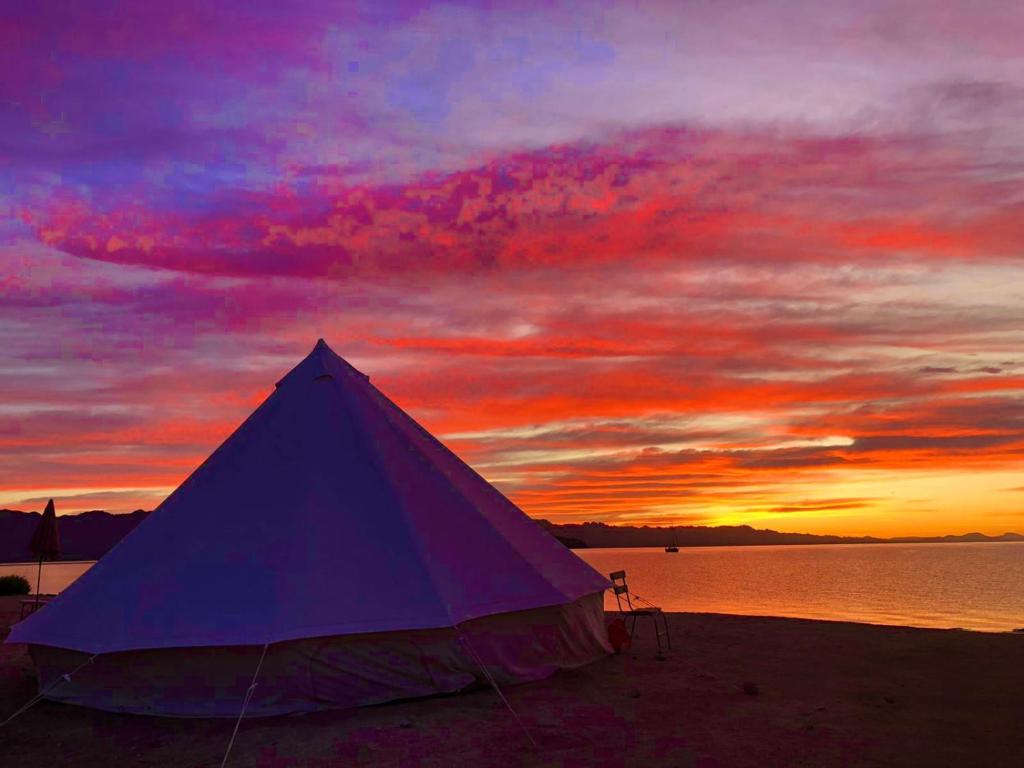This image captures a serene scene at either a beach or lake in the early evening. Dominating the foreground is a large, triangular tent with a blue top and dark-colored base. Right in front of the tent, there is a small chair facing the water, which gently ripples under the evening sky. The sky is a stunning gradient, starting with purples and dark clouds at the top, transitioning through pinks, deep fire orange, and finally to yellow as it approaches the horizon. This vibrant display of colors reflects on the water, giving it a dull orange hue. In the middle of the image lies the calm body of water, framed by an outline of hills in the distance. To the left lower part of the image, the tent rests on dark gray ground. The overall scene is accentuated by the setting sun, surrounded by a blend of orange and yellow light. There is a boat gently drifting on the water, adding to the tranquility of the scene.